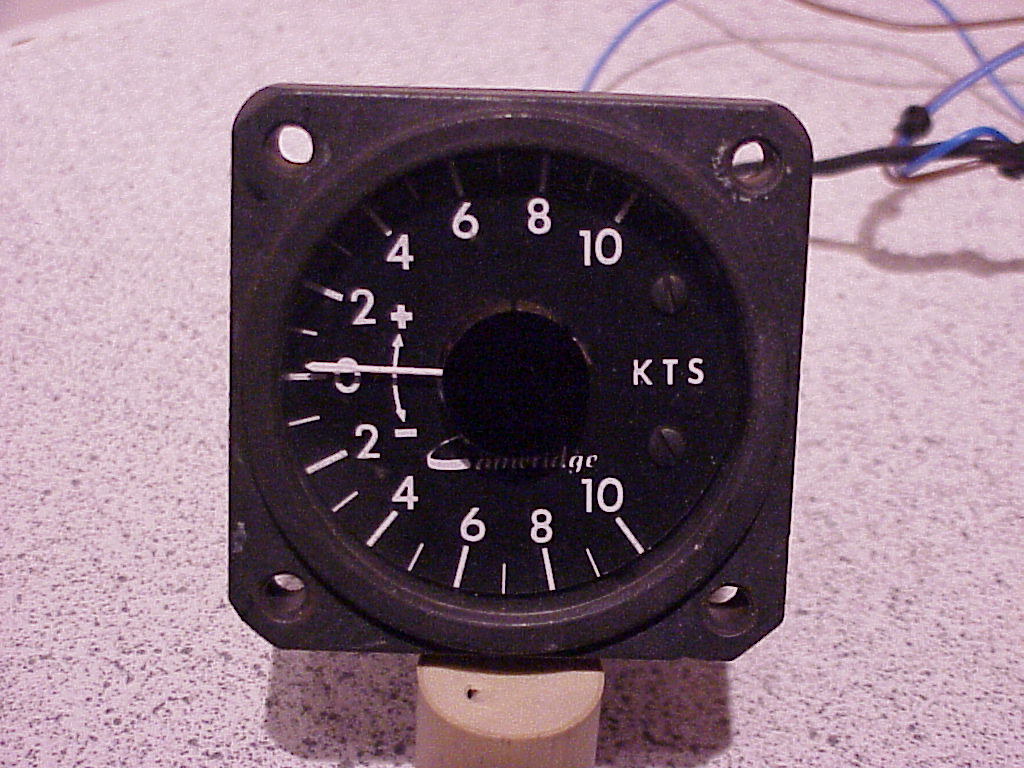The image features a square gauge with a numerical scale prominently displayed against what appears to be a concrete surface. The gauge is loose and not secured, as evidenced by the empty screw holes in each corner. The numerical scale is arranged in a circular manner, starting from the top and progressing counter-clockwise with values: 10, 8, 6, 4, 2, 0, -2, -4, -6, -8, and -10. A noteworthy detail is the section on the right side where the numbers between 10 and -10 are encircled, framing the letters "KTS."

At the center of the gauge is a single, white metal pointer, resembling a clock hand, aligned with the scale to indicate readings. The pointer, numbers, and all visible lettering on the gauge are in white, ensuring clear contrast against the background of the gauge.

In the backdrop, two wires—one blue and one black—are visible, adding an element of utility and function to the scene. The gauge rests upon a round base, possibly made of wood or cork, further emphasizing its provisional placement and the overall utilitarian context of the image.